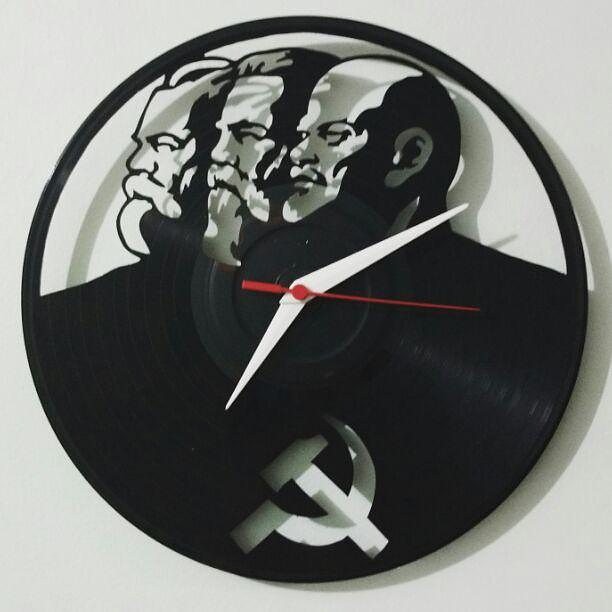This photo features a modern clock crafted from a vinyl record against a white background. The clock has mid-century modern white hands and a red second hand, displaying a time of about 7:12. In the lower section of the record is a carefully cut-out symbol of a hammer and sickle, emblematic of Soviet Russia. Above this, etched into the top half of the record, are detailed silhouettes of three historical figures, side by side. From right to left, they are likely Vladimir Lenin, Joseph Stalin, and another Soviet leader, possibly Leon Trotsky. The figures are arranged in a stoic, almost solemn demeanor. The juxtaposition of the modern clock design with these significant symbols of Soviet history adds an intriguing contrast, making the piece both an artistic and historical statement.